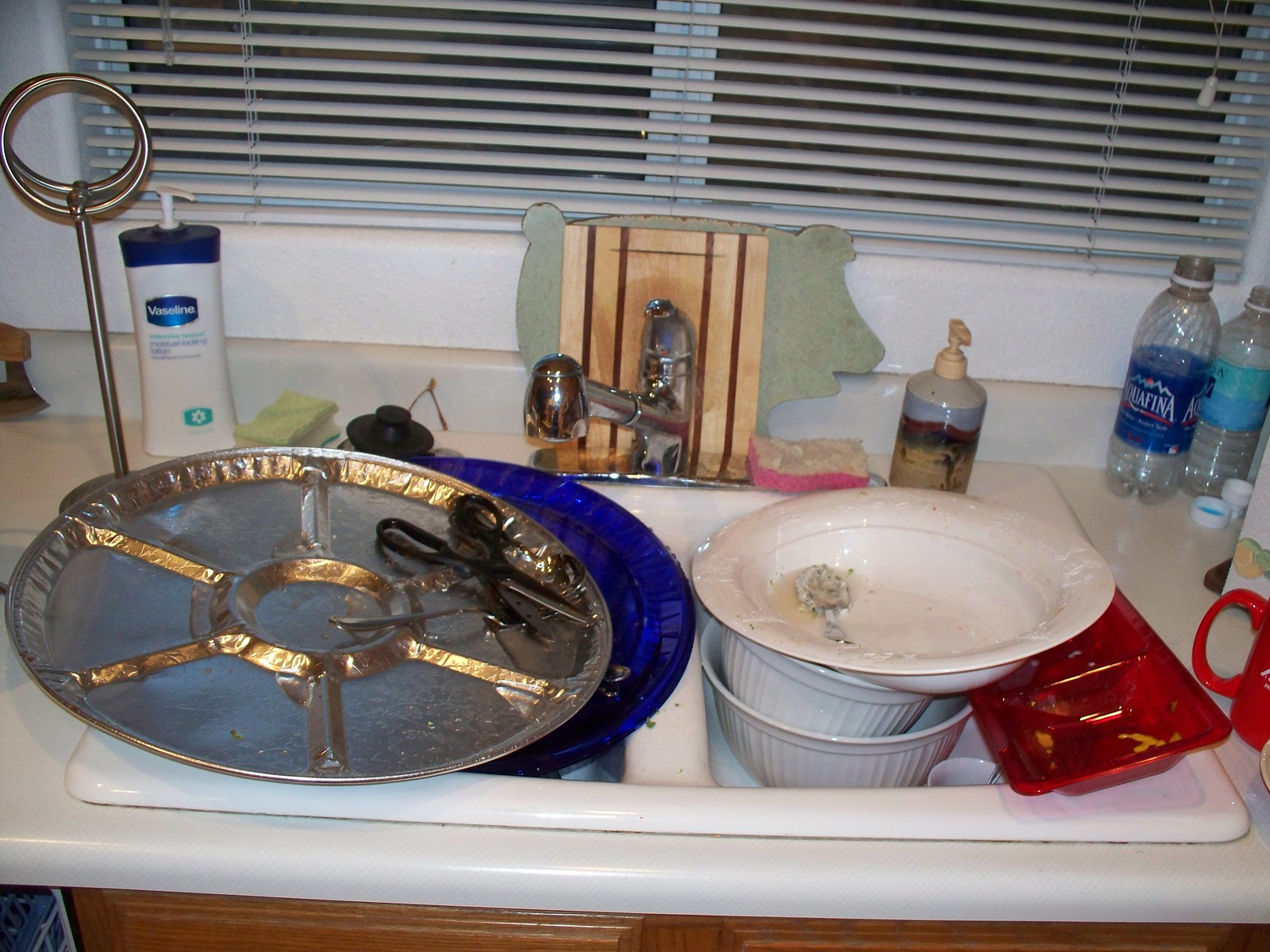A photograph showcases a bustling kitchen sink filled with dirty dishes. The white enamel sink, characterized by its double basin with a raised central divider, features a sleek silver faucet with a single handle for controlling water temperature. Surrounding the sink is a collection of cleaning essentials, including a scrub pad, a sponge, a soap dispenser, and a water stopper for the basin. Additionally, a second scrubber and a bottle of lotion are placed nearby. A brass rod with rings, likely intended for holding towels, stands prominently from its base beside the sink. The cluttered sink itself is packed with various kitchenware, including numerous white porcelain bowls, a red plastic tray, and an array of utensils, such as scissors and a spoon. The topmost bowl displays remnants of food, hinting at the aftermath of a recent meal preparation.